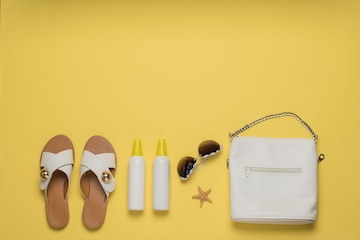In a neatly arranged and highly organized photograph set against a simple yellow background, five distinct beach items are displayed along the bottom portion of the image. On the bottom left corner, there is a pair of white flip-flops adorned with a light brown leather sole and a gold button accent on the straps. Next to the flip-flops, two small, bright white spray bottles with yellow tops stand side by side. To their right, almost centrally placed in the photograph, is a pair of aviator sunglasses with dark lenses and a gold frame. Just below the sunglasses lies a brown starfish, adding a touch of natural oceanic beauty to the scene. Completing the lineup on the far right is a chic white leather purse with a chain handle, featuring a zipper on the front and another zippered section on the side. This meticulous arrangement highlights a selection of essential beach items, designed with elegance and simplicity in mind.